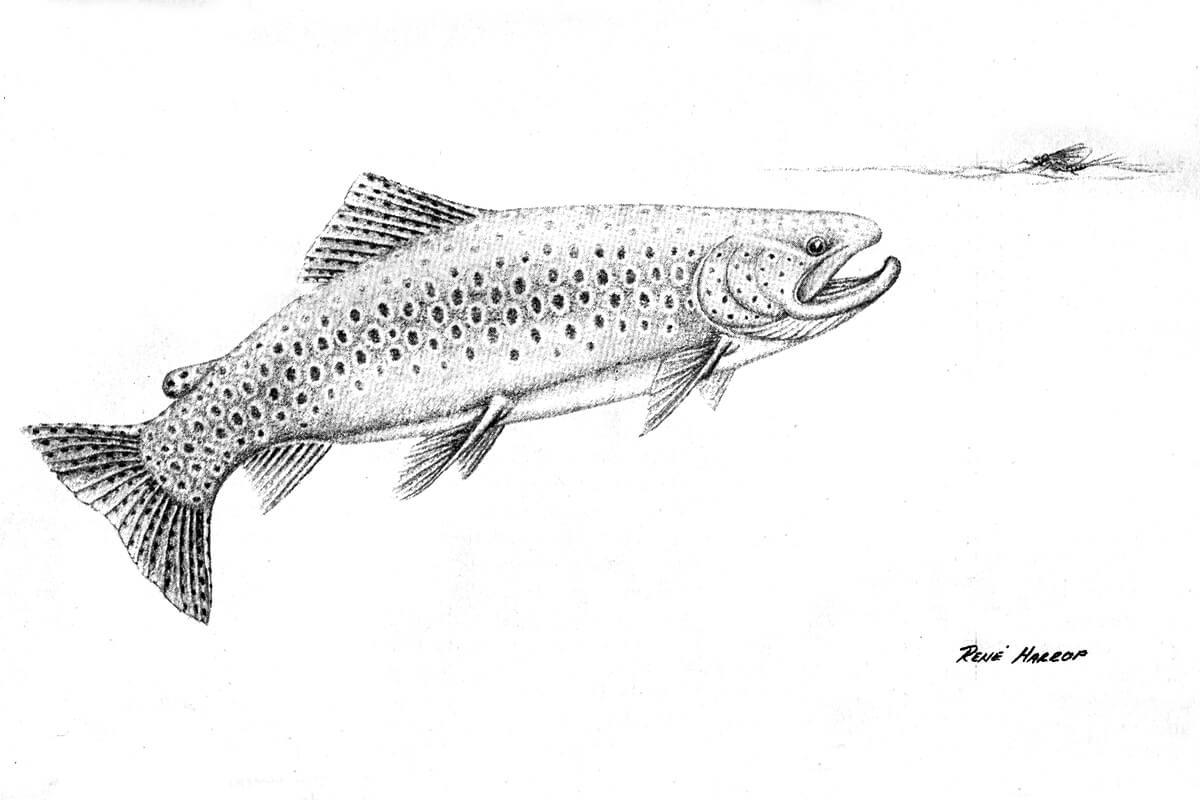This pen and ink drawing by artist Rene Harrop illustrates a dramatic scene of a spotted bass poised to strike an insect resting on the surface of the water. Rendered entirely in black and white with nuanced gray shading, the image captures the tension of the moment with striking detail. The fish, depicted in profile, faces right with its mouth open, eyes locked on its prey—a delicate insect resembling a mosquito. The illustration is set against a stark white background, which emphasizes the intricate details of the bass and the calm surface of the water. The composition is rectangular, with the tail fin of the bass positioned just below the center left and the head near the center slightly to the right. Harrop’s meticulous use of ink brings the scene to life, highlighting the textures and patterns on the fish’s skin and the subtle ripples on the water’s surface.